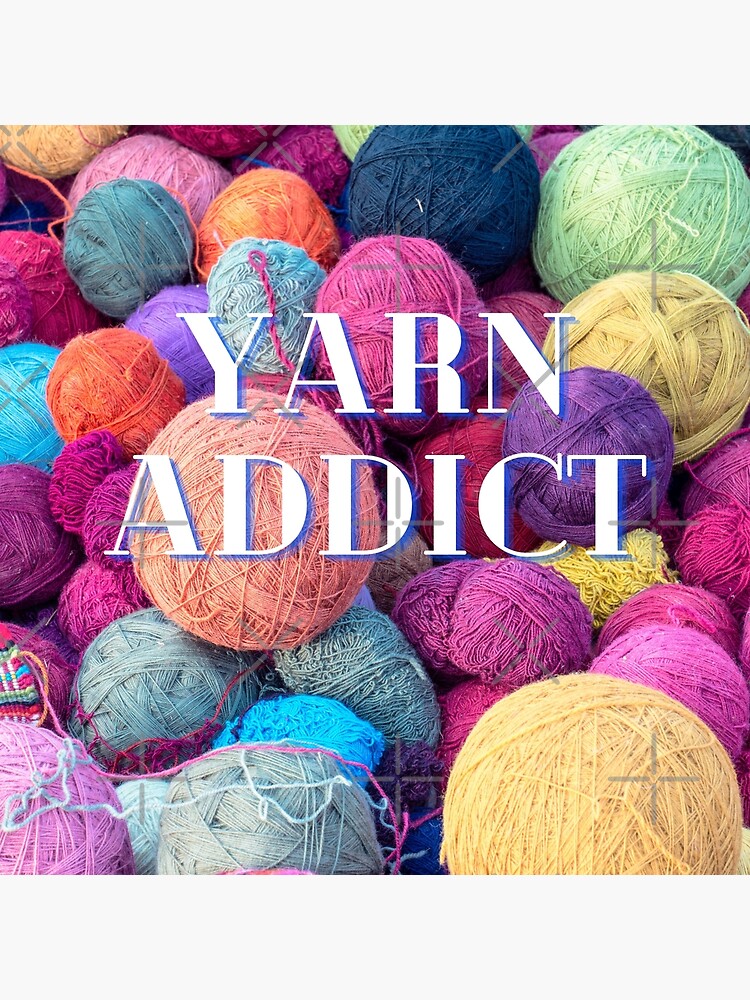This square photograph is packed with a vivid assortment of yarn balls in diverse colors, ranging from various shades of purple, green, and blue, to oranges and multiple tones of yellow. Some balls are loosely wrapped, others are tightly coiled, and a few even take on an oblong, log shape reminiscent of how they appear for sale in stores. Yarn strings freely dangle and overlap, giving the scene an authentic, used feel. Overlaid in bold white block capital letters, the text "YARN ADDICT" reinforces the theme. A subtle grid pattern featuring plus and X shapes faintly adorns the background, adding a textured layer to the vibrant composition.